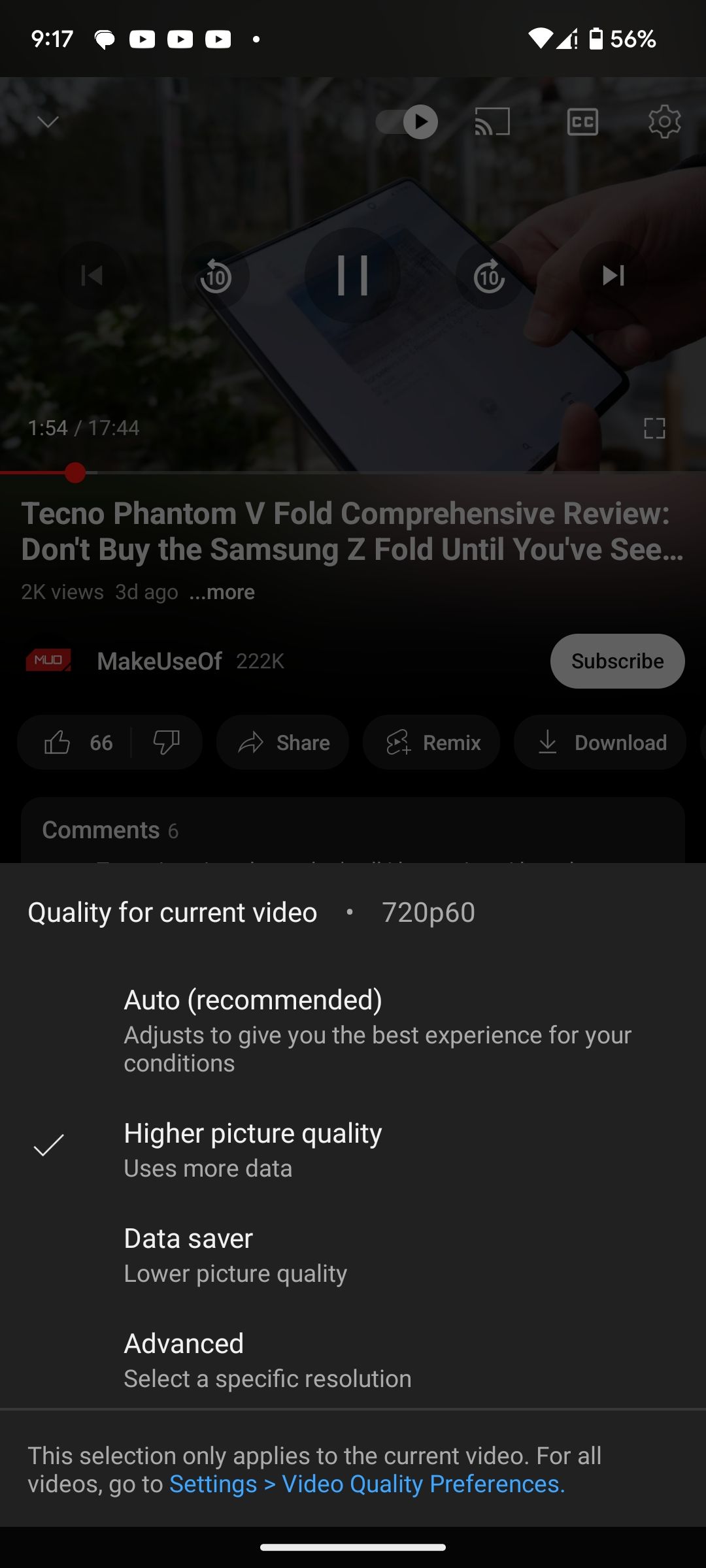The image depicts a cell phone screen with a black or deep slate gray background, displaying various elements. The time on the device is 9:17, and there's an active text message. Three YouTube video thumbnails are visible, alongside icons indicating Wi-Fi connectivity and a battery level of 56%. All information is displayed in white text on the dark background.

In the top right corner of the screen, a toggle switch is positioned to the right. Below it, partially obscured by a gray film, is a paused YouTube video with icons for cast, closed captions, settings, and playback controls. These controls include options to rewind 10 minutes, fast forward 10 minutes, and skip to the end of the video. The progress bar indicates the video is at 1:54 of 17:54 minutes.

The video title is "Technobantam 5 Fold Comprehension Review - Don’t buy the Samsung Z Fold until you've seen this," with 2,000 views accumulated over the last three days. The channel, "Make Use Of," has 222,000 subscribers, and there's a white 'Subscribe' button. The video has garnered 66 likes, and there are buttons for dislike, share, remix, and download, along with six comments.

The video quality is set to 720p60, with an auto-recommended setting to ensure optimal streaming based on current conditions, and the 'higher picture quality' option is selected.